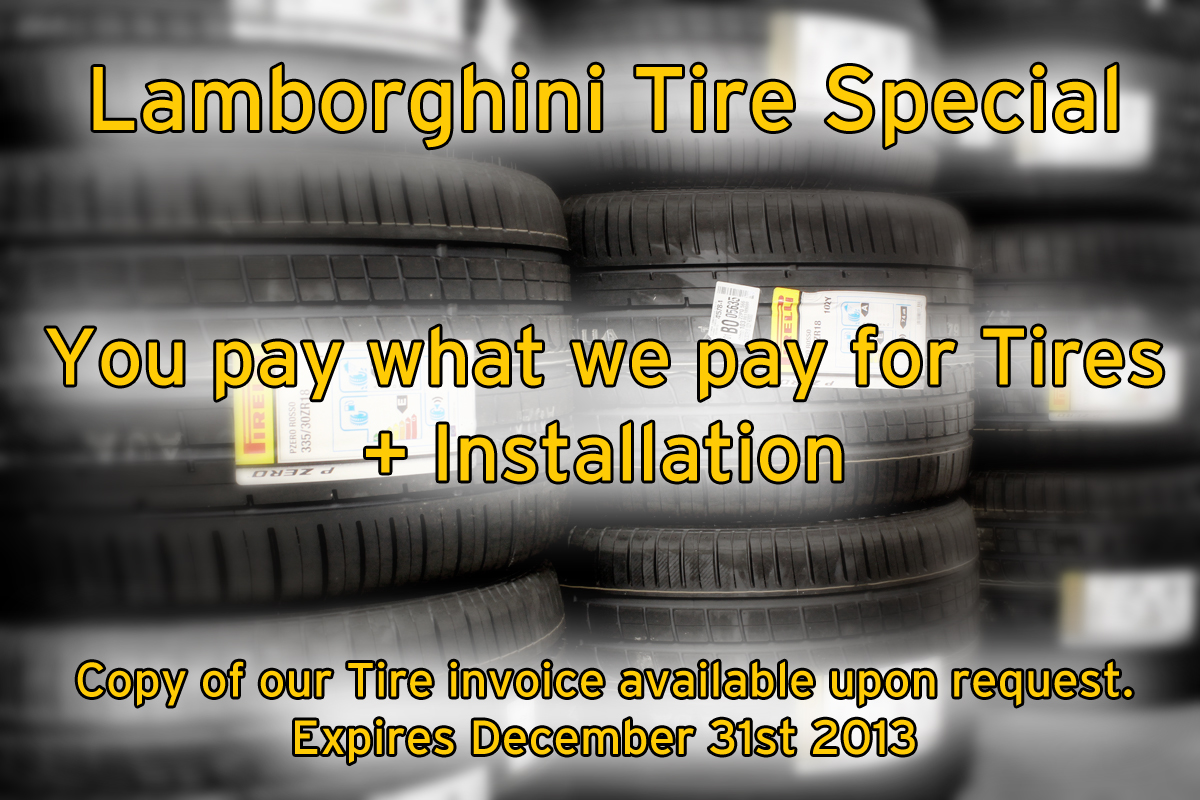The image is a horizontal rectangle showcasing a digital ad with a stylized photograph of neatly stacked tires in three rows. The photo, primarily in shades of black, gray, and white, has a slightly blurred background to emphasize the text. Overlaid on the image is bright yellow text with a black outline and a soft white blur around it. The text, positioned in three sections, reads: "Lamborghini Tire Special" at the top, "You pay what we pay for tires + installation" in the center, and "Copy of our tire invoice available upon request. Expires December 31st, 2013" at the bottom. The tires in the background, around six or seven in total, feature white labels detailing their specifications, although the specifics are obscured by the overlaying text and blur effect.